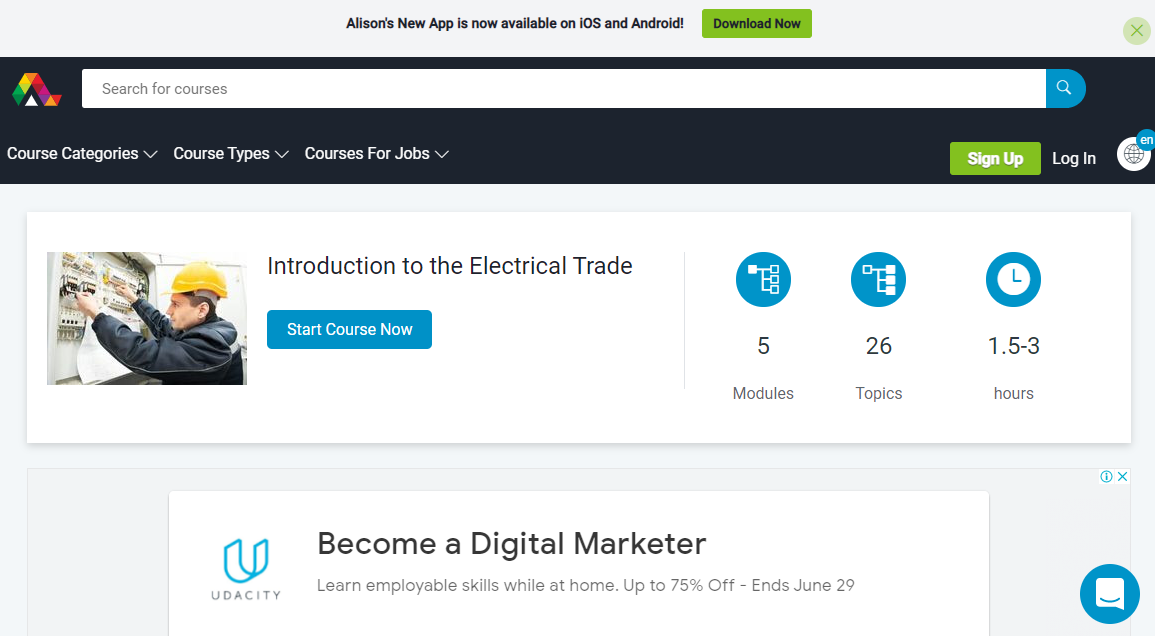**Descriptive Caption:**

The screenshot is from a website's course section. On the left side of the page, there are navigational sections labeled "Course Categories," "Course Types," and "Courses for Jobs." Dominating the central area, a prominent bar featuring a small image of a man working on an electrical box is present. Adjacent to this image, a headline reads "Introduction to the Electrical Trade." Below this heading, there is a blue button labeled "Start Course Now." To the right of the button, three icons are displayed with numbers beneath them: 5, 26, and 1.3, representing "Modules," "Topics," and "Hours," respectively. Further below, another featured course box highlights "Become a Digital Marketer." This section promotes learning employable skills from home and offers a discount of up to 75% that ends on June 29th.